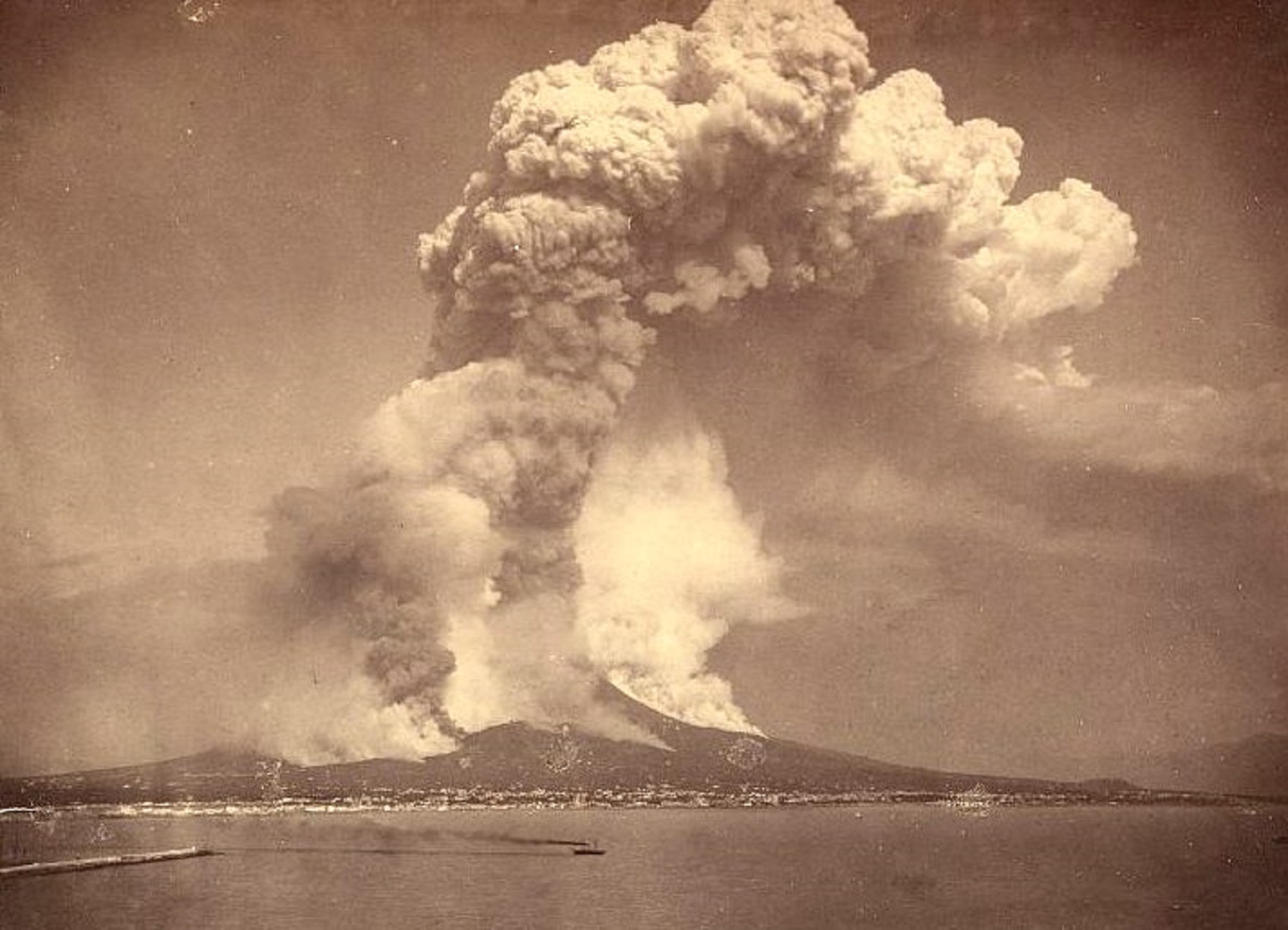The image depicts an old, sepia-toned historical photograph capturing a dramatic volcanic explosion. At the center of the photograph, a massive column of smoke rises from the volcano, resembling giant cauliflower clouds, while various streams of smoke billow outwards from the eruption. The photo, slightly grainy and blurry, adds to its vintage and historical feel. The volcano is situated on an island, surrounded by water, emphasizing its isolated violence. Far from the chaotic scene of the eruption, several ships, including a tugboat with black smoke emanating from its engine, can be seen traversing the waterfront, providing scale and context to the immense plumes dominating the image. The photograph, marked by white spots due to its age, captures the eruptive moment with a sense of severity and power.